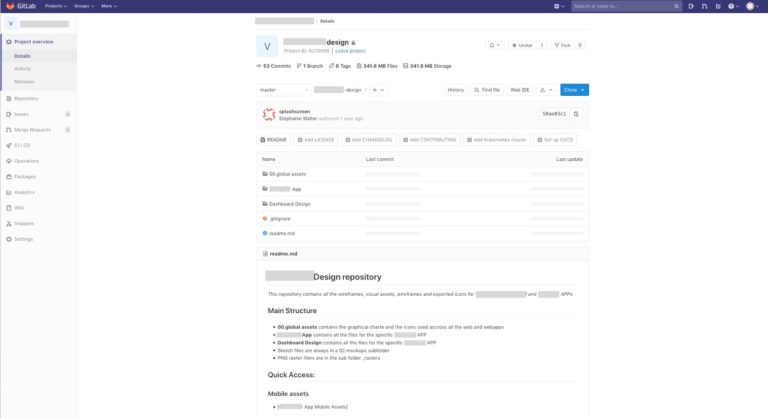A screenshot of what appears to be a GitLab interface, with various elements partially obscured or difficult to read, is displayed. In the upper left-hand corner, a small-text logo, possibly reading "GitLab" or "GiftLab," is enclosed within a purple border. The top navigation bar includes links labeled "Product," "Services," and "More," alongside a search bar situated in the upper right-hand corner.

On the left-hand sidebar, categories listed are "Product Overview," "Details," "Activity," and "Preferences." Some subcategories are visible, such as "Analytics," "Wikis," and "Settings," while others are difficult to discern.

The main content area features a white background with some gray blocks intentionally obscuring certain sections. At the top, under the label "Details," a hidden block of text is marked by a gray overlay. Adjacent to a "V" logo, the text "Design" is visible, along with an indication of "53 comments" and "one search."

Below this, the content includes a readme file section. Key headings within it include "Design Repository," "Main Structure," "60 Global Assets," "App," "Dashboard Design," "Quick Access," and "Mobile Assets." Much of the remaining text in this section is not clearly legible.